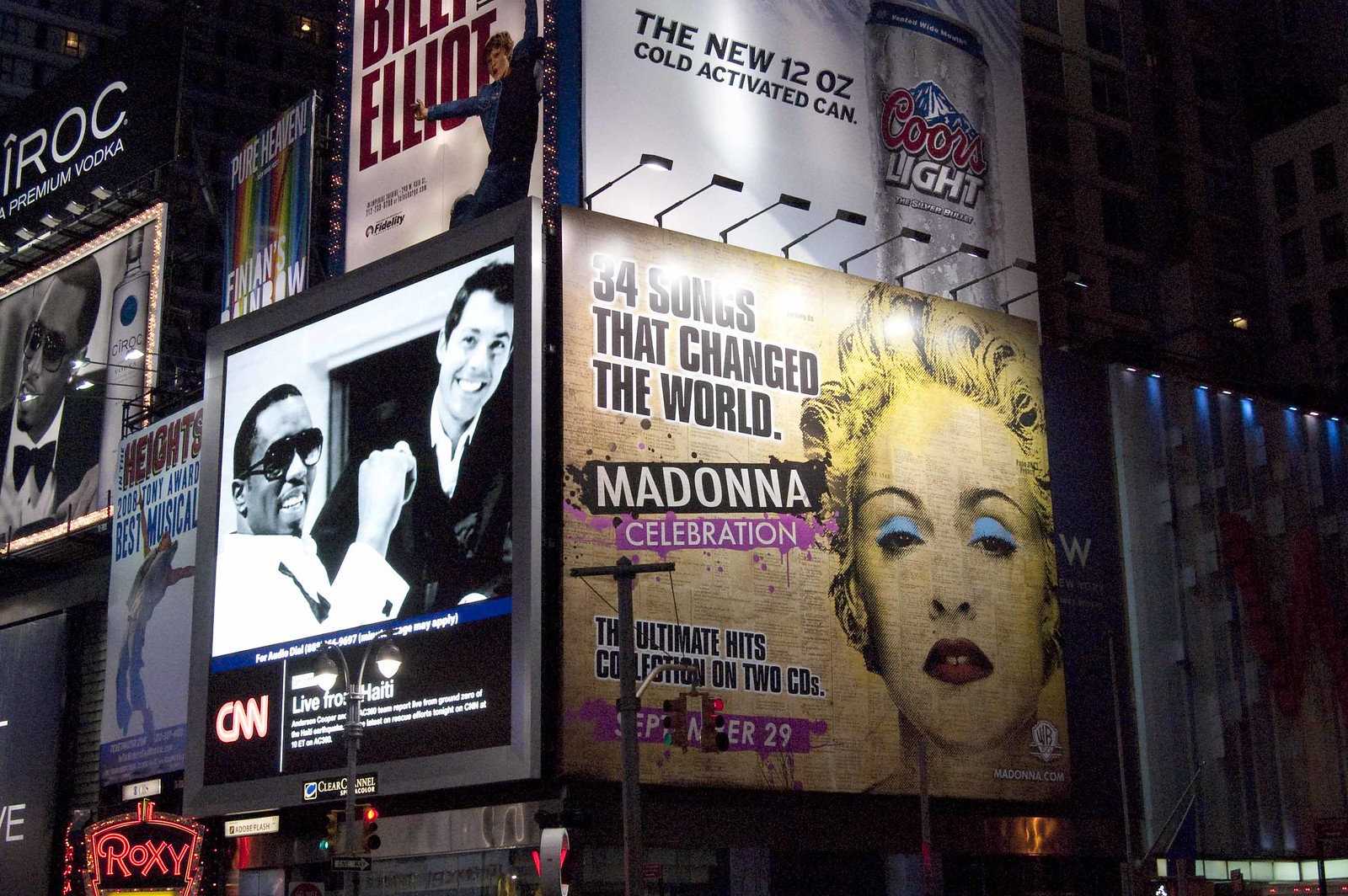The image depicts a bustling corner billboard in what appears to be Times Square, New York City. At the top left, an advertisement for Billy Elliot is prominently displayed. Below it, a striking black-and-white photo of two celebrities announces "CNN, Live from Haiti," accompanied by several lines of white text. To the right, an eye-catching ad for Coors Light showcases their new 12-ounce cold-activated can. Directly beneath this, the billboard highlights a major promotion for Madonna's Ultimate Hits collection, which includes "34 Songs That Changed the World." Madonna, with blonde hair, is featured wearing vivid blue eyeshadow, red lipstick, and yellow makeup. Her lips are slightly parted, set against a cream-colored background. The detailed portrait of Madonna draws attention to the advertisement that reads, "Madonna Celebration, Ultimate Hits Collection on Two CDs, September 29th." Among this visual tapestry of ads, the left-hand side of the billboard also features promotions for IROC Premium Vodka. Several skyscrapers and the partial exterior of a wall frame the scene, capturing the vibrant and dynamic marketing ambiance typical of a major urban center.